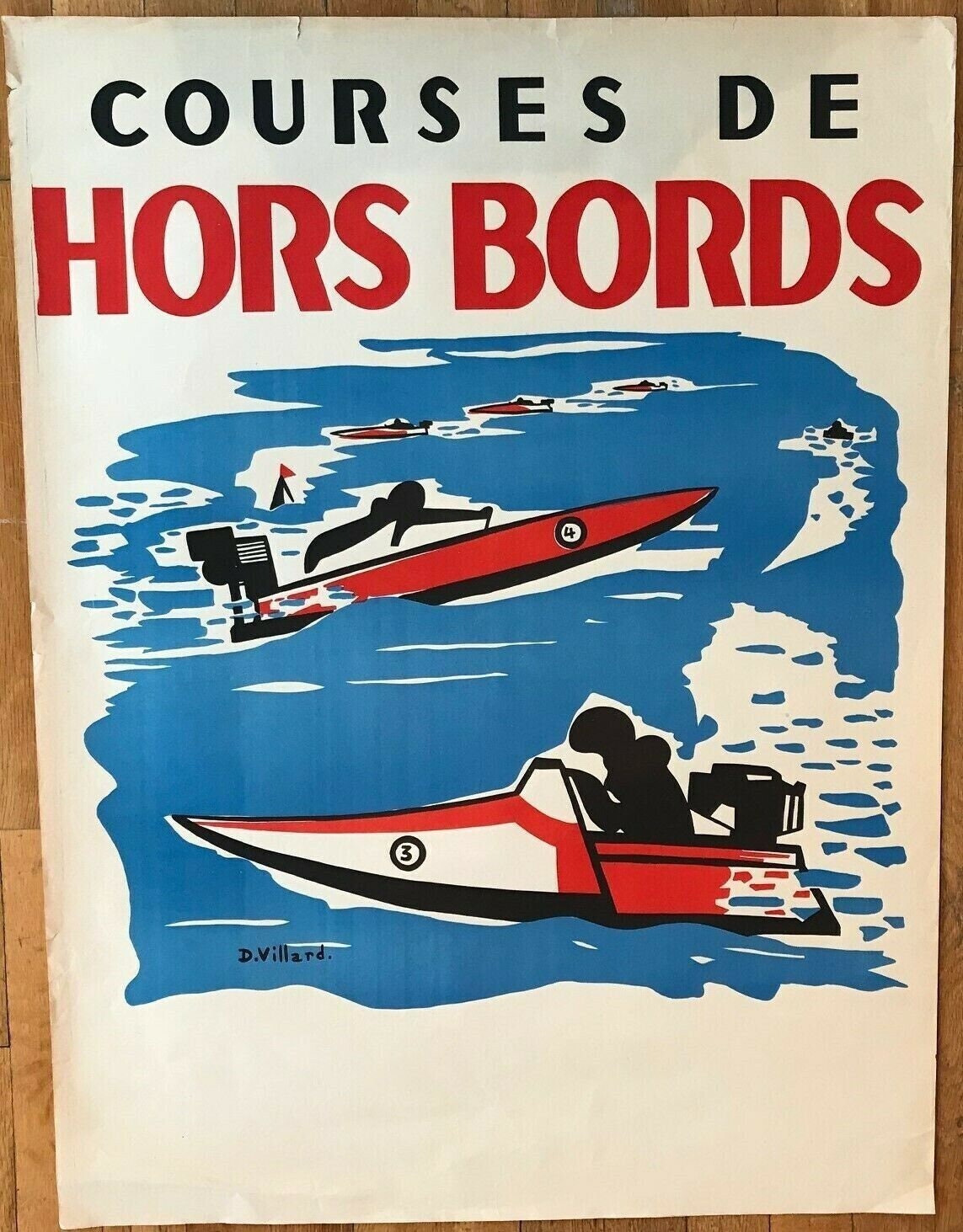The image showcases an aged and weathered poster displayed against a tan wood background. The poster itself is printed on white paper and features a vibrant blue splotch representing water at its center. This body of water is populated with several speed boats and jet skis, each leaving white wakes in their path. The prominent foreground includes a red speed boat with a white stripe and the number three, equipped with a black engine and a simplistic black figure in the boat's seat. Another red boat with a black engine and a distinguishing white circle with black trim on its side is seen in the background, alongside three smaller red boats. There also appears to be a small dog in the water. The header text at the top of the poster, displayed in a foreign language presumably French, reads "Courses des Horreboards," with the top line in black and the bottom line in thicker red block letters. The name "de Villard" is penciled in at the bottom left corner of the poster.